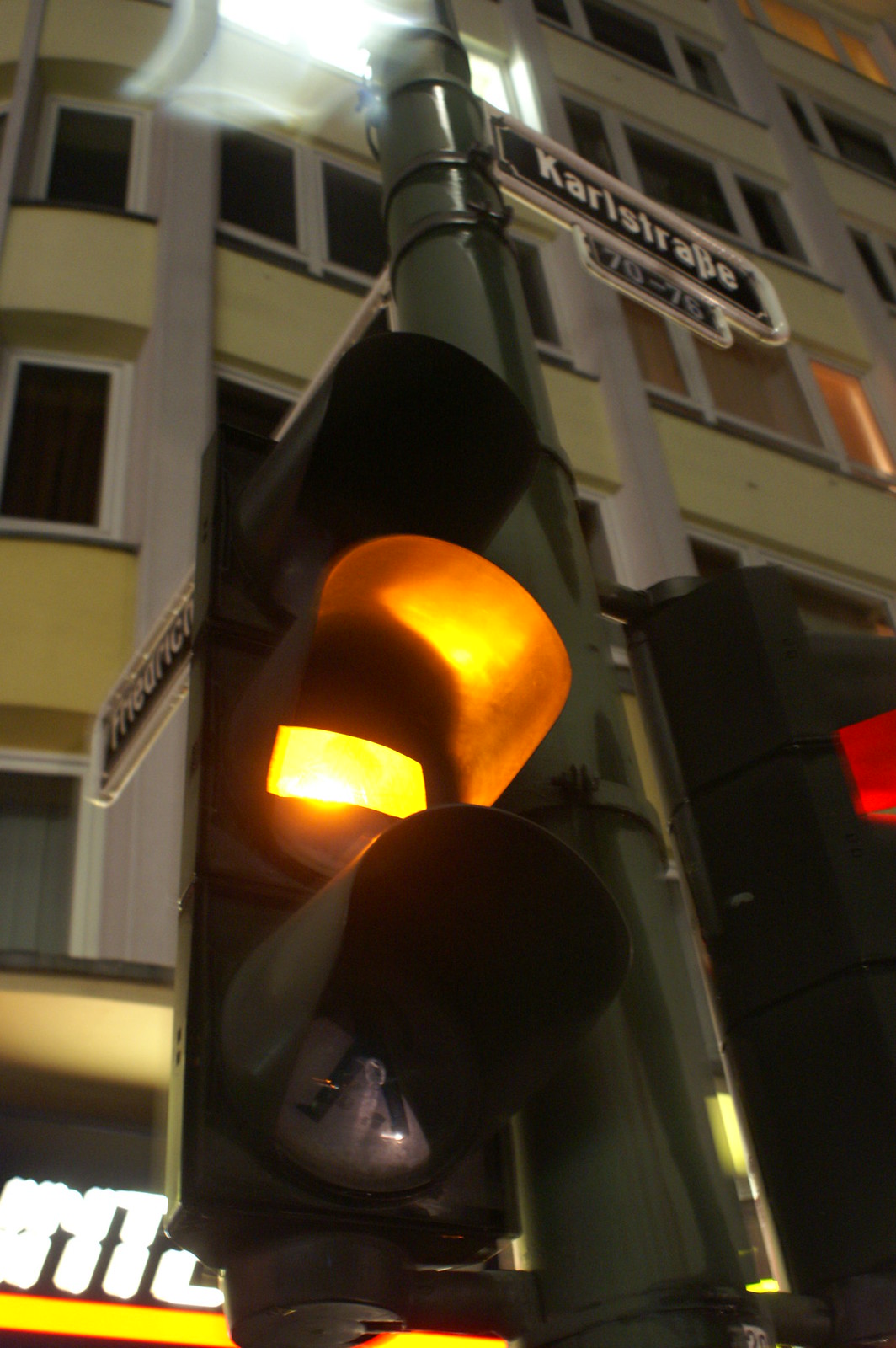In this nighttime photograph taken in a German city, a dark green pole supports two traffic lights and several directional signs. The nearest traffic light in the center prominently displays a glowing yellow rectangle, while a partially visible traffic light on the right side shows a red signal. Above these lights, a black and white street sign reads "Karlstraße 70 to 76." The background features a multi-story apartment building painted in light yellow with white-trimmed windows and vertical cement pillars. At the base of the building, a white and yellow sign indicates a business located behind the traffic signals. The scene is bathed in artificial illumination, emphasizing the urban nightscape.